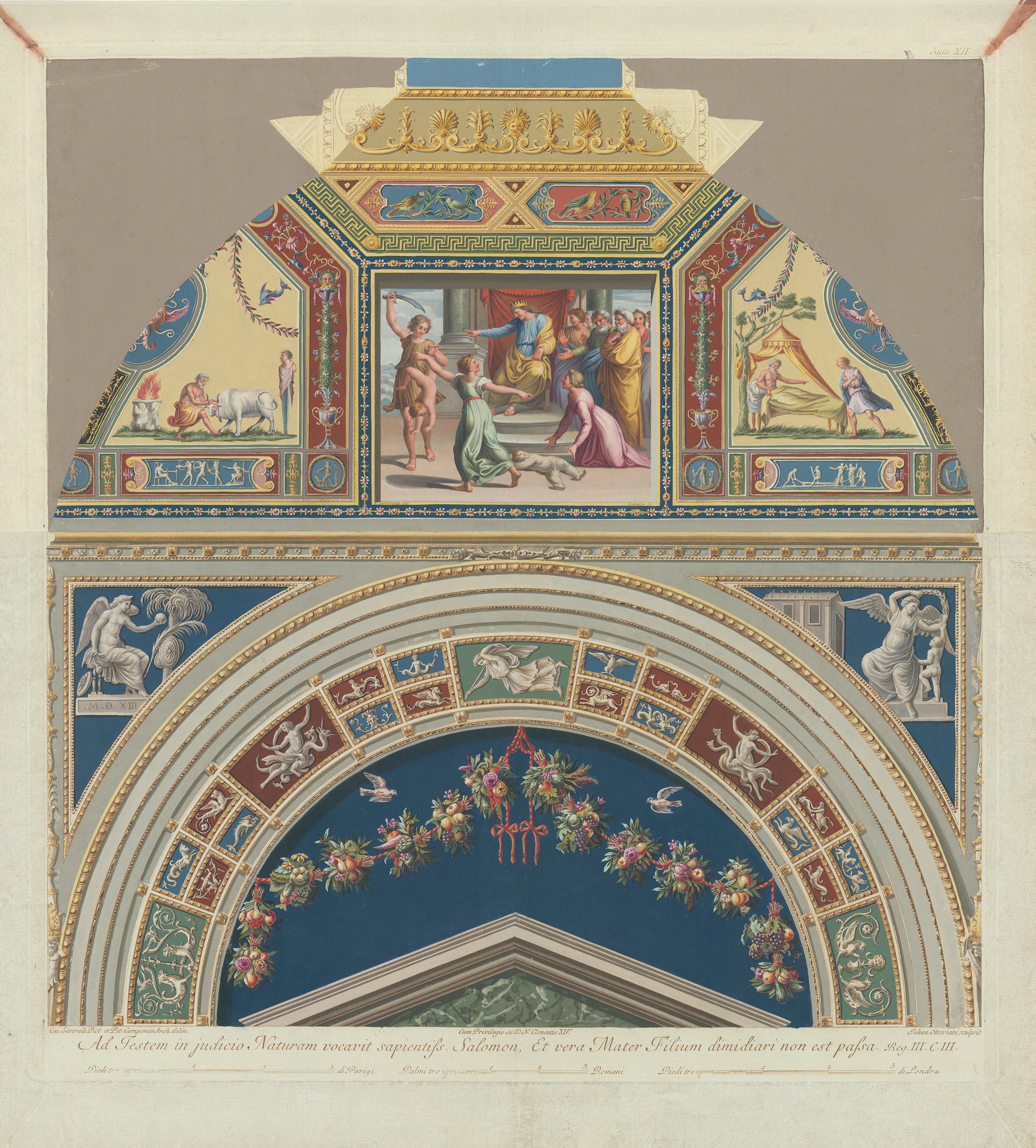The image depicts an intricate and richly detailed piece of 14th-century artwork, possibly from a museum or historical textbook. It features an array of vibrant colors, including green, red, and blue, achieved with high-quality inks that suggest the artisan might have been sponsored by aristocrats. The art is framed with curved corners and adorned with Latin text at the bottom. Central to the piece, there are figures in religious or holy garb, including a crowned man, elder men and women, and a woman carrying a child and a sword, highlighting ancient beliefs and possibly biblical scenes. Cherubs and angels populate the painting, surrounded by dancing figures, flowers, garlands, and a golden outline. Notable details include a person holding a goat in the top left and another person lying in bed at the top right, adding to the depiction’s elaborate scene of people engaged in various activities, reflective of medieval religious and cultural practices.